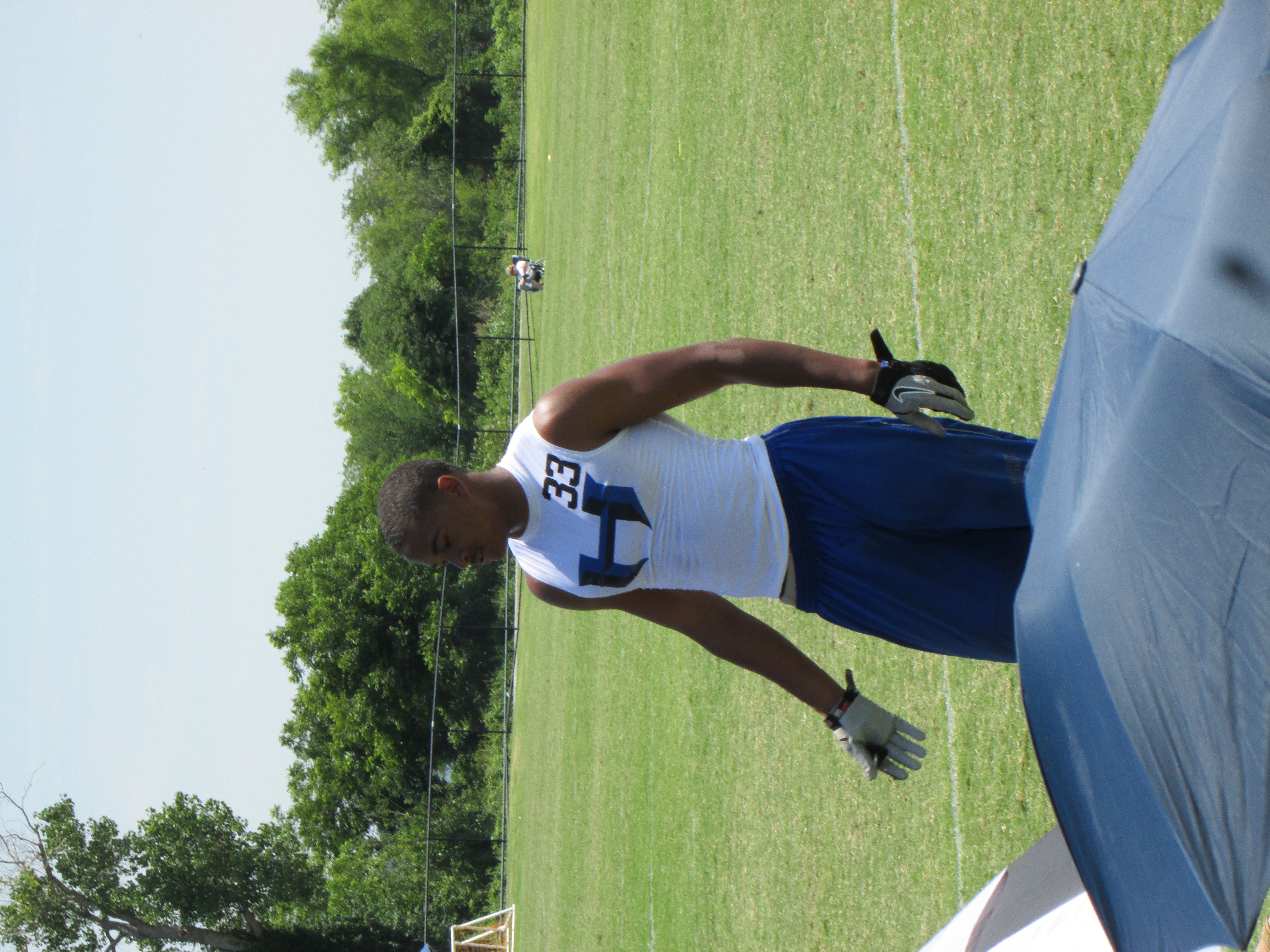This image captures a sideways-angled photo of a young, muscular black male athlete standing on a large grassy field surrounded by greenery, shrubbery, and a chain link fence. The sky is clear and blue, indicating it is a sunny day. The man has short, dark hair and is dressed in a tight, sleeveless white t-shirt featuring a large, stylized letter "H" on the front and the number "33" in black on the left side of his chest. He is also wearing navy blue shorts, gray and black Nike gloves, and standing with his arms at his side. In front of him on the grass lies a navy blue umbrella that is open. To his right, there is a second soccer goal visible, and a person can be seen in the background, possibly cutting the grass.